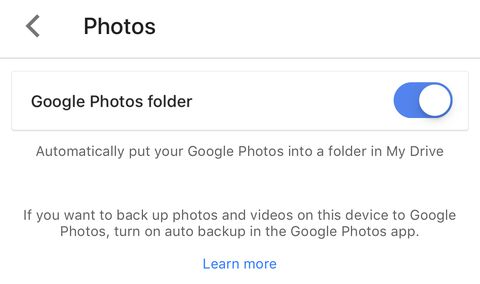The image is a screenshot captured on an iPhone, displaying a section of the Google Photos settings interface. The background is predominantly white. In the top-left corner, there is a back arrow icon followed by the word "Photos" in black text, indicating navigation within the photos section. Beneath this, there is a long white rectangle with the label "Google Photos folder" on the left side. Adjacent to this label on the right side is a blue checkbox. Below the rectangle, a line of black text reads, "Automatically put your Google Photos into a folder in My Drive." Further down, in smaller black text, it advises, "If you want to backup photos and videos on this device to Google Photos, turn on auto backup in the Google Photos app." At the bottom of the frame, there is a blue button labeled "Learn more." The entire screenshot is surrounded by gray border lines, delineating different sections of the interface. The overall composition is simple, with a primary focus on the textual information and interface elements highlighted within the screenshot against a minimalist white background.